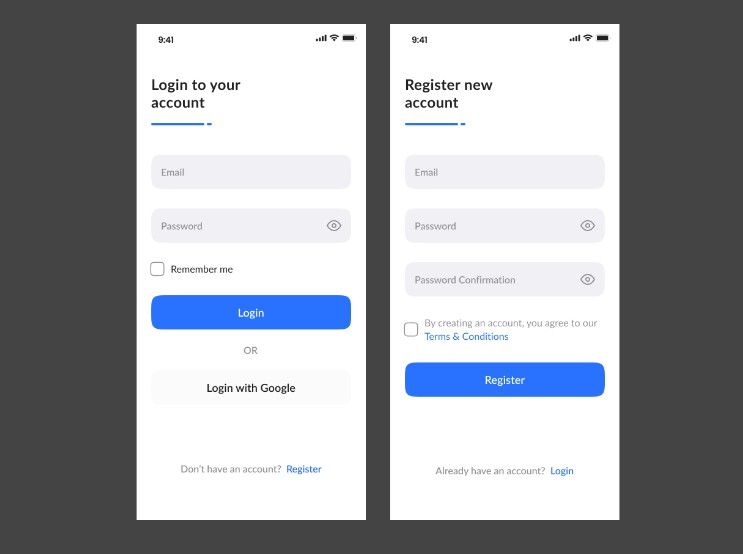The image features a gray background, resembling the size of a computer screen. Set against this background are two vertical, white sections that resemble either pages or phone screens. Both sections display "9:41" in the top left corner, accompanied by icons for battery charge and Wi-Fi connection on the top right.

The left section is titled "Log into Your Account." Beneath the title, there is a field for users to enter their email address, followed by a password entry box. Below the password box, there are options for the user to remember their login details via a "Remember Me" checkbox. Further down, there are two buttons: one reads "Log In" and the other offers an alternative login method with "Log In with Google."

The right section is titled "Register New Account." Similar to the left section, it has fields for entering an email address and a password. Below the password box, a note reads, "By creating an account, you agree to the Terms and Conditions." Finally, a button labeled "Register" allows users to complete their new account registration.